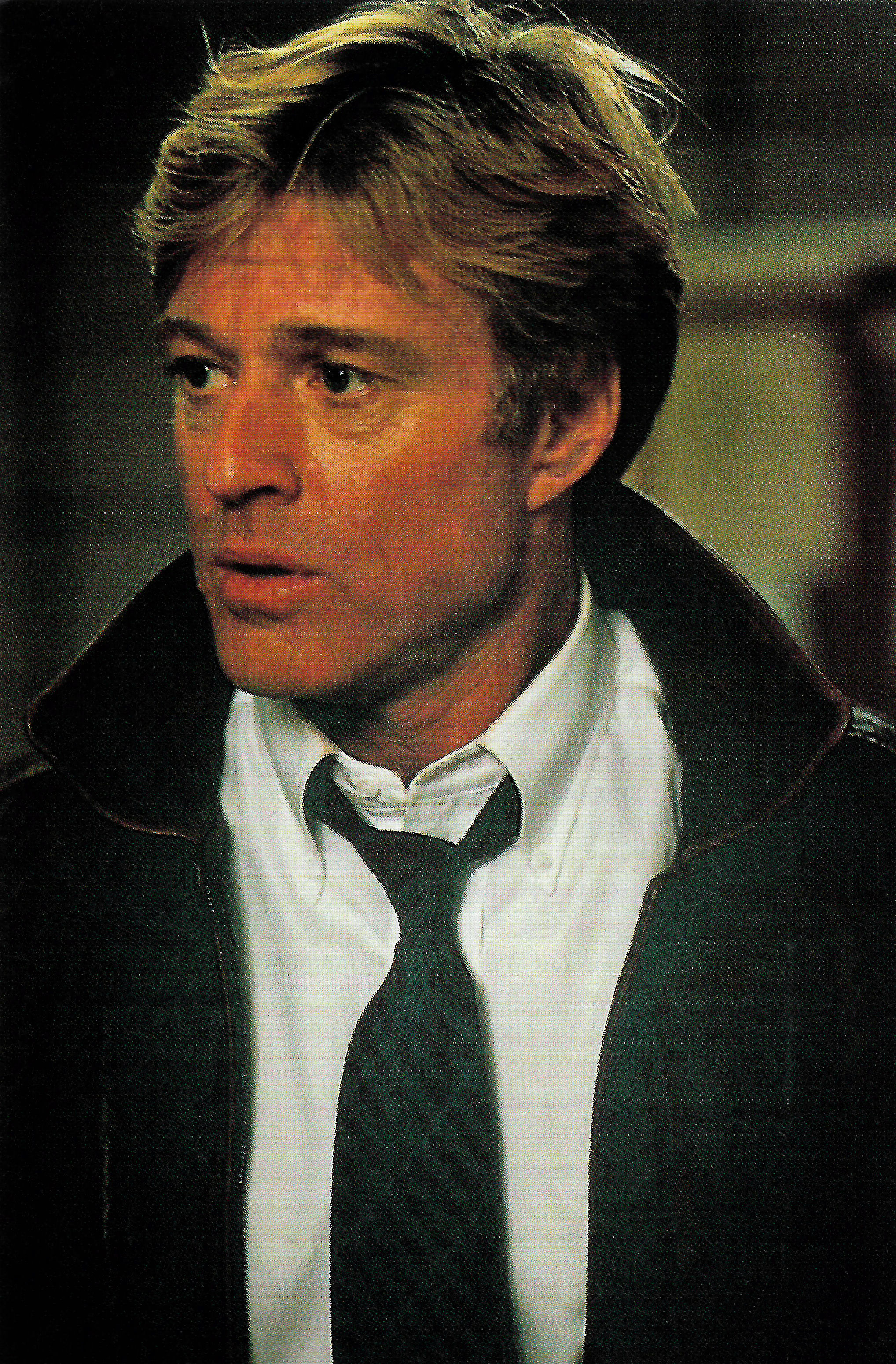The image, captured indoors, appears to show a scene reminiscent of an older movie or a TV show, perhaps displayed on a screen. The top portion of the picture features grainy tones of black and gray, with hints of white and yellow shading on the right-hand side. The background is somewhat fuzzy and indistinct, primarily brownish in color.

Dominating the foreground is a famous actor, though his name escapes recollection. He has strawberry blonde to bleached blonde hair with subtly visible brown roots. His hairstyle includes sideburns extending down his cheeks, parted towards the left and combed to the right, with a slightly wavy and slicked-over texture.

The attire of the actor is notable: he wears a white button-down shirt, the top button undone, paired with a loosely knotted blue tie. Over this, he sports a black jacket, which is unbuttoned, and the collar is stylishly spiked upwards. The actor's face focuses in the distance towards the left side of the image, capturing a pensive expression. A distinguishing feature is a small mole or birthmark near his nose. The image conveys a vintage and reflective ambiance through its visual elements and the actor's contemplative pose.